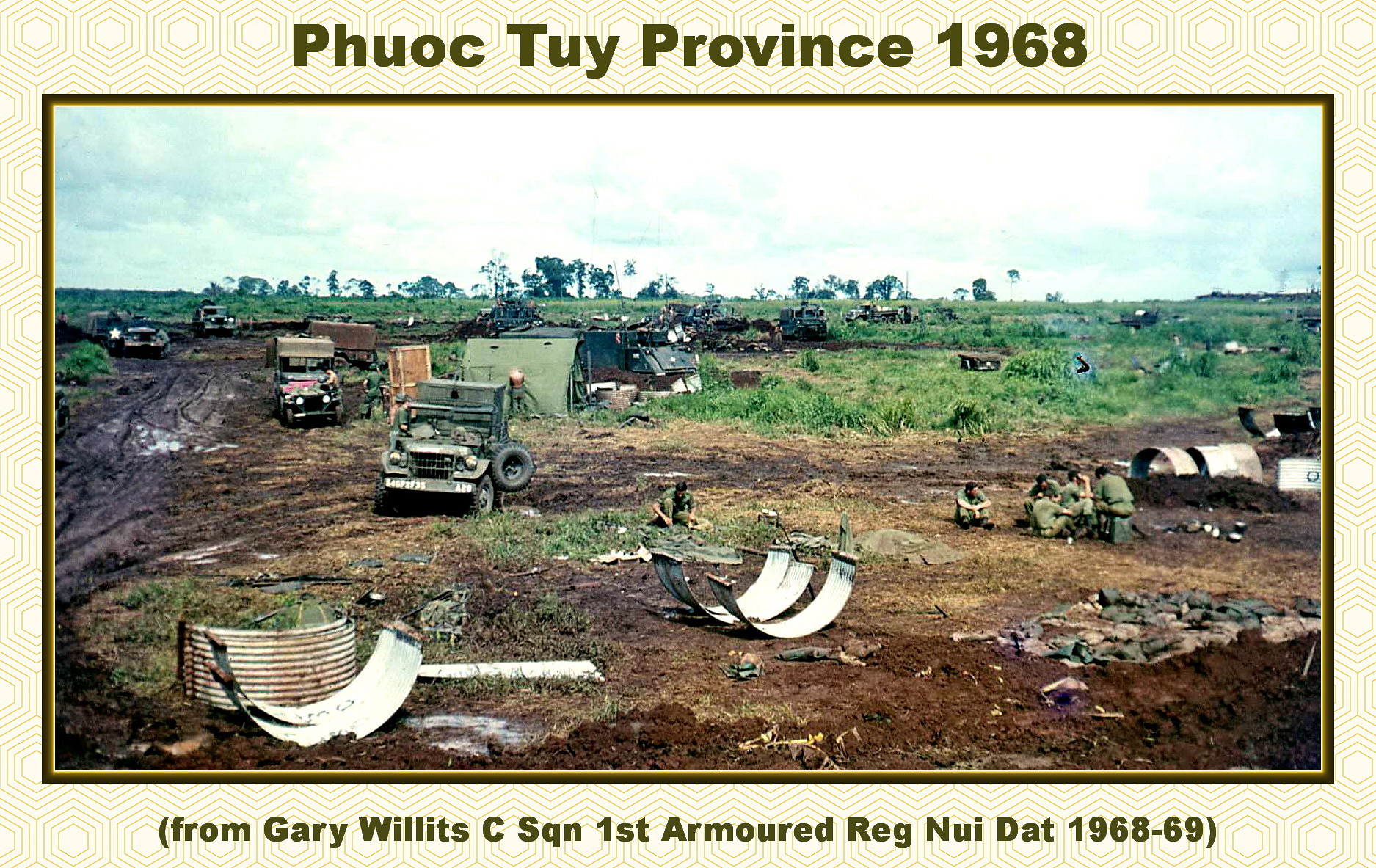This detailed military photograph, framed with a tan border, bears a header reading "Phuoc Toi Province, 1968," and is attributed to "C-Squadron 1st Armored Regiment, Noonday, 1968-69," signed by Gary Willett. Captured within the province during the Vietnam War, the image depicts a muddy roadway lined with parked military vehicles, each carrying various cargoes. To the right, a cluster of soldiers, clad in military uniforms, sit on the ground near a pile of stones and scattered curved metal sheets, suggesting remnants of broken equipment. Surrounding this scene are several military tents and an array of bags and equipment strewn across the area, indicating a temporary encampment. The backdrop features a flat, grassy field dotted with numerous army trucks and other vehicles, all beneath a cloudy sky which enhances the somber atmosphere of this war-torn landscape.